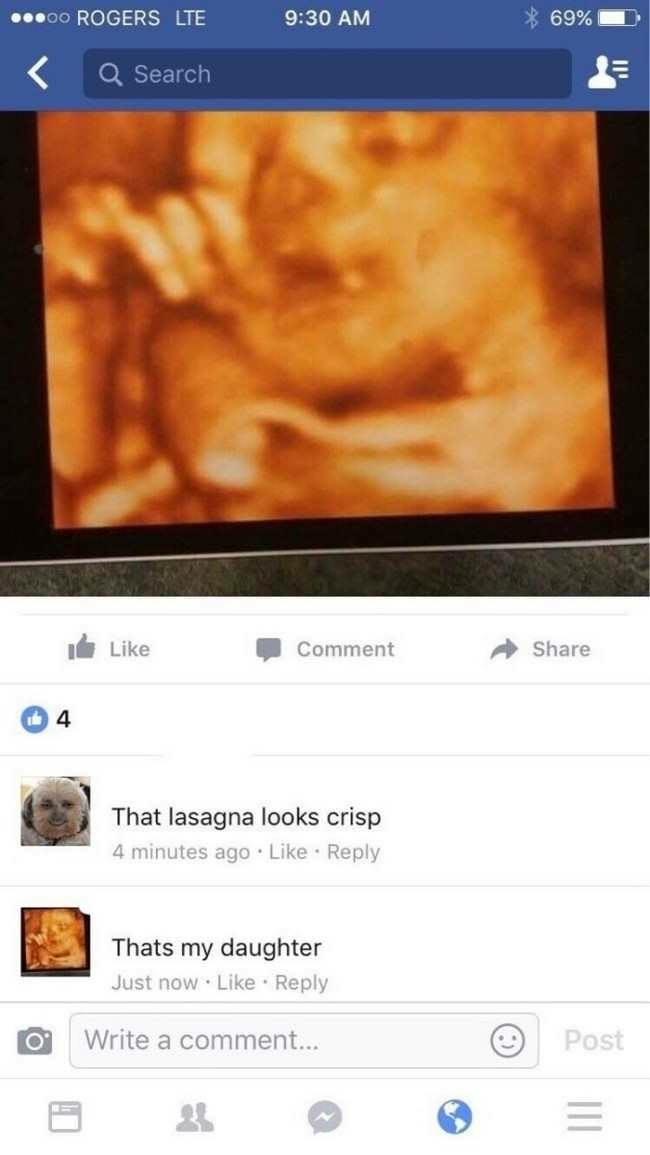This is a detailed screenshot of a Facebook post, depicting an ultrasound image of a developing baby, but the image is indistinct, featuring orange and brown hues that some might mistake for lasagna. At the very top, the phone's notification bar shows "Rogers LTE," the time at "9:30 a.m.," a 69% battery life indicator, and the Bluetooth symbol. Just below, against a blue background, there is a search bar and a settings button. The post includes interactive Facebook elements like "like," "comment," and "share" buttons, showing it has received 4 likes. Below the image, a humorous comment exchange is visible: one user remarks, "that lasagna looks crispy," to which the poster replies, "that's my daughter." Further down, the interface offers options to write a comment, post, add a photo, and other settings.